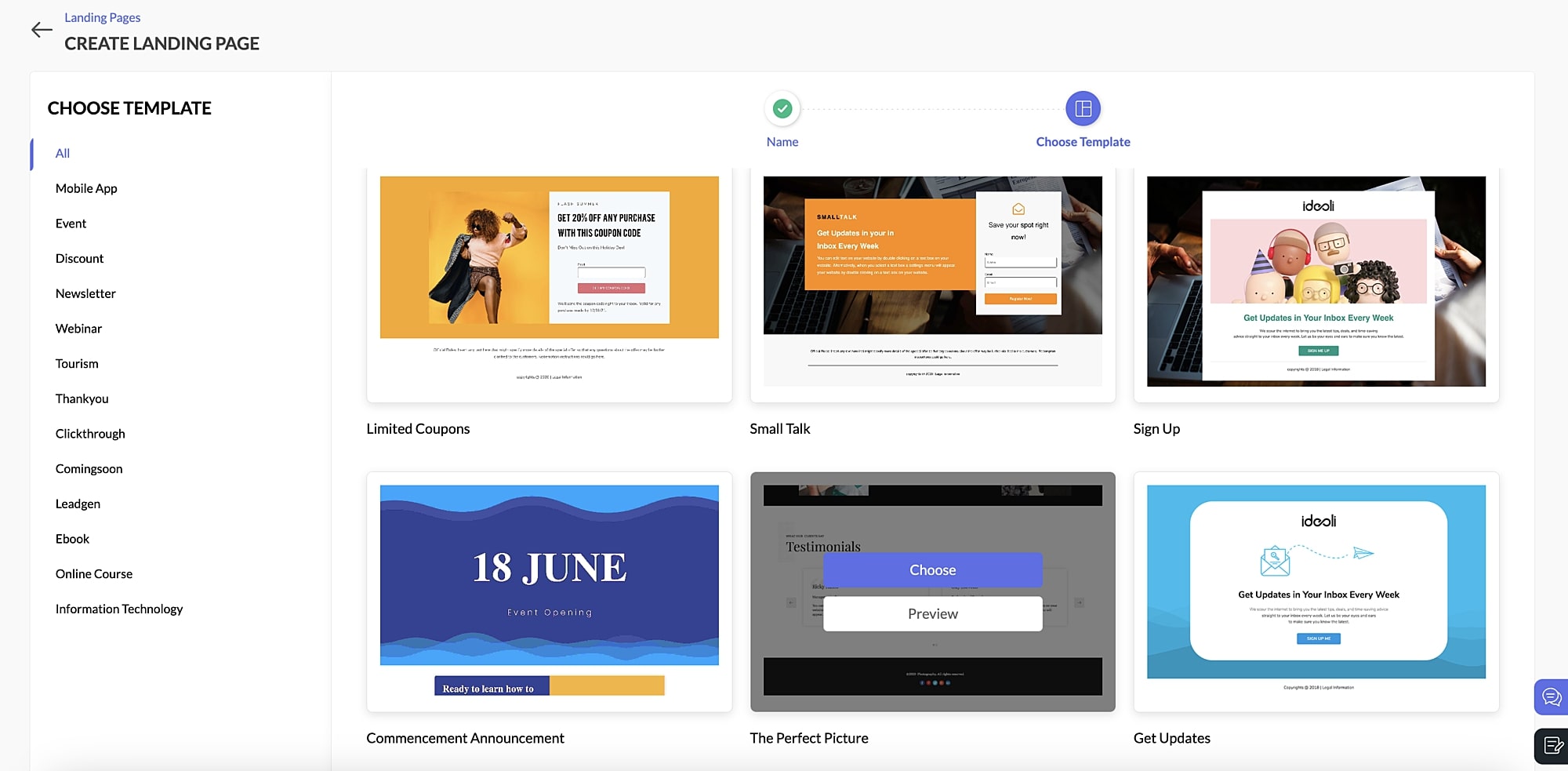The image showcases an interface of a website builder specifically focused on creating landing pages. In the top left corner, there is a label that reads "Landing Pages" followed by a back arrow. Below this, in bold black letters, it says "Create Landing Page." Further down, another bold black heading states "Choose Template."

The main section features various template options listed in a structured layout. The templates are organized in two rows, with three templates in each row. From left to right, the first row includes templates labeled "Untitled," "Email," and "Sign Up." The second row features "Commencement Announcement," "The Perfect Picture," and "Get Updates."

Additionally, at the top of the center section, there is a prominent new button indicated by a green arrow. Positioned above the templates, the "Choose Template" section has a blue button, drawing attention to the selection process. The overall design is clean and user-friendly, facilitating easy navigation and template selection for users looking to create landing pages.